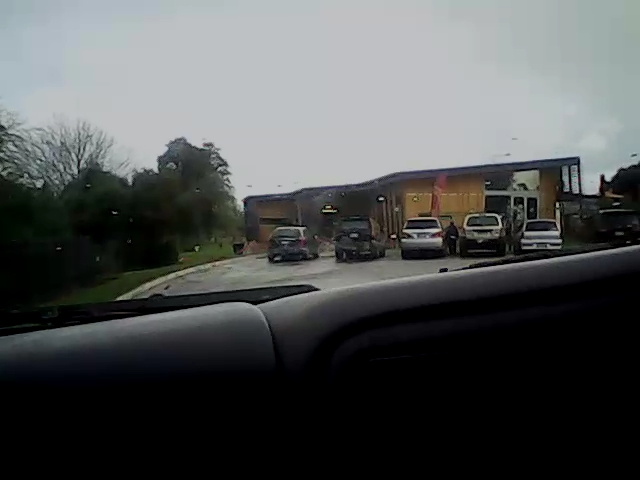Photographed from inside a vehicle, the image captures the scene outside, focusing on an unidentified commercial building. The building features a flat roof that slightly angles upward and has silver-bordered entrance doors. The setting is somewhat obscured by raindrops on the windshield, indicating recent rain and lending a gray tint to the sky. 

In the foreground, five cars are distinctly visible in the parking area, with the possibility of a sixth vehicle somewhat obscured. To the left of the building, a variety of trees populate the landscape, including dense green foliage alongside taller, leafless trees. The overall atmosphere is one of a rainy day at what could be a business or retail establishment, detailed but slightly blurred through the lens.